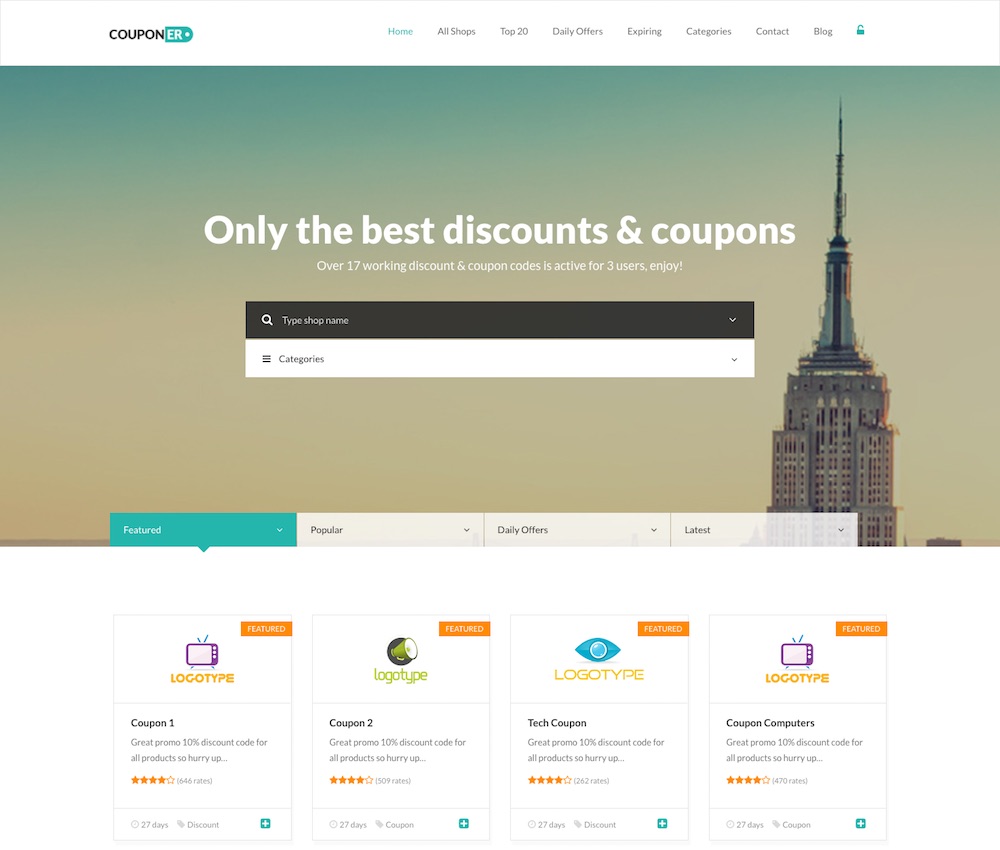In the upper left corner, the word "COUPON" is displayed in black, fully capitalized, followed by the letters "ER" inside a green circle. Below, in green text, the navigation options "Home," "All Shops," "Top 20," "Daily Offers," "Expiring," "Contact," "Categories," and "Blog" are listed. Adjacent to these options is a green lock icon. 

The background transitions from blue at the top to a light brown or beige at the bottom. Centered prominently are the words "Only the Best Discounts and Coupons." To the right, there's a tall building resembling a space needle with a thin, pointed top. 

A search bar is provided with an input field, and beneath it, the word "Categories." Further below, tabs in a green box display "Featured," "Popular," "Daily Offers," and "Latest." 

At the bottom, there are four coupons displayed:
1. Coupon one with a specific logotype.
2. Tech coupon with an image of a purple television set; below it, the logotype is in yellow letters, and "Coupon Computers" is written in black letters.